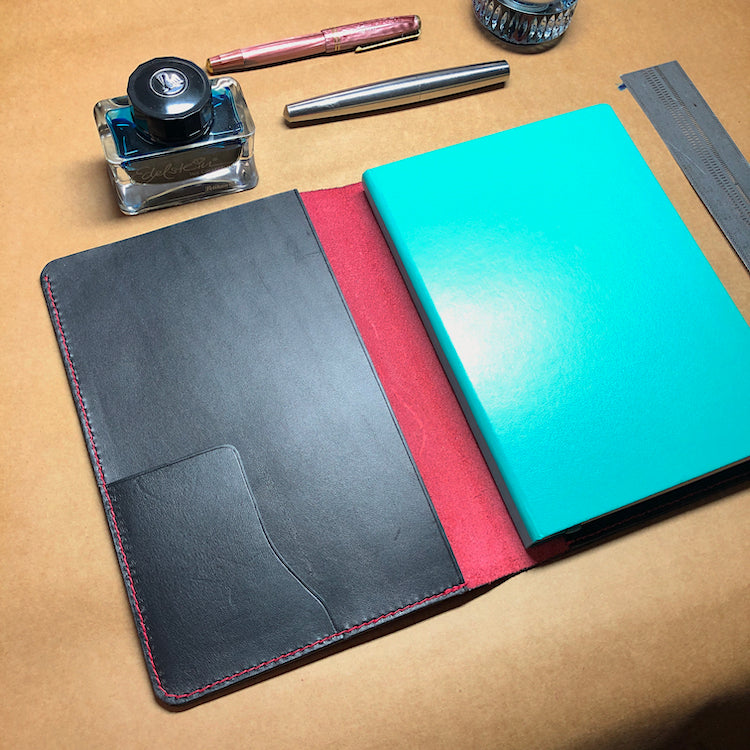This photograph captures an organized, aesthetically pleasing workspace centered around a high-quality journal. At the heart of the image lies a blank sky blue notebook, encapsulated by an elegant black leather cover which is open to reveal its striking red inner lining and a practical internal pocket. Flanking this setup is a collection of sophisticated writing instruments; notably, there are what appear to be two high-end fountain pens situated near an ornate inkwell, with an additional inkwell possibly visible in the top right corner of the frame. To the immediate right of the notebook, a sleek metal ruler is neatly positioned. The desk itself is a neutral beigey-brown color, perhaps leather-topped or wooden, contributing to a refined and minimalist ambiance. This well-arranged space suggests a perfect environment for jotting down notes, lists, or journal entries.